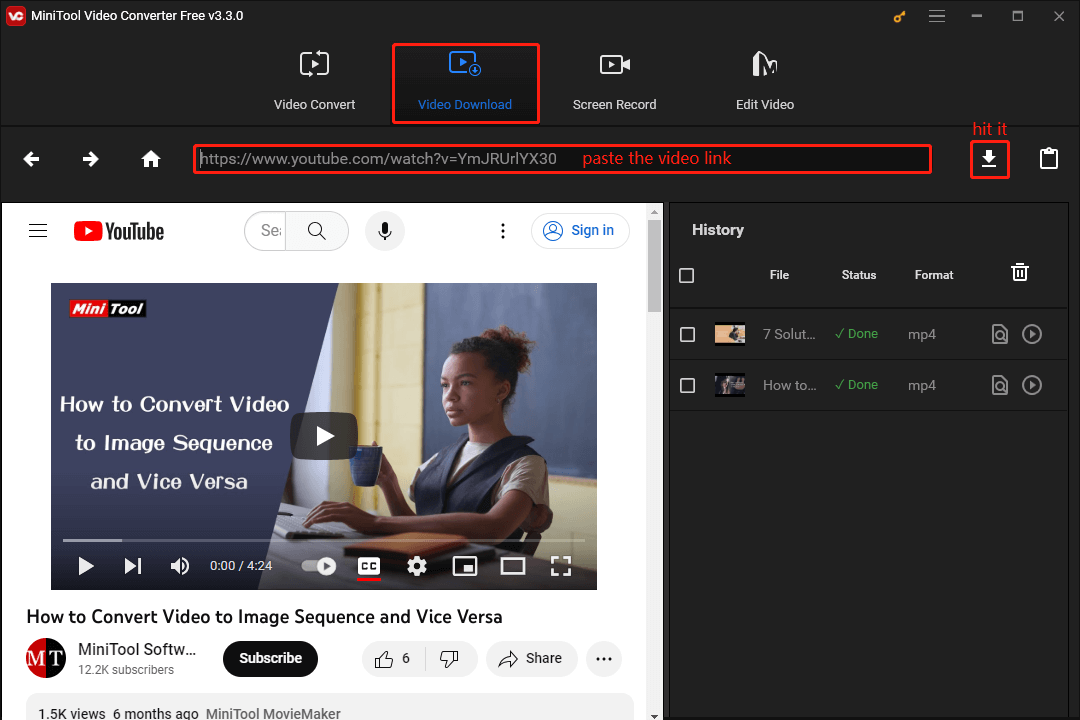The image has a rectangular orientation with its longer side extending from left to right. It predominantly features a black background. At the very top, a red box contains the white letters "VC" and is followed by the text "MiniTool Video Converter Free Version 3.3.0" in white. To the top right, standard control icons for minimizing, maximizing, and closing the window are present.

In the next section, four options are listed horizontally: Video Convert, Video Download, Screen Record, and Edit Video. The "Video Download" option is highlighted with a red-lined box, and its font is blue, while the other options are in white.

Moving further down, a navigation bar resembling a URL page appears. It includes left and right arrows, a Home icon, a URL input box outlined in red, and a 'Hit It' button on the far right.

Below this, on the left side of the screen, there is a YouTube sign-in page displaying a video titled "How to Convert Video to Image Sequence and Vice Versa." A large Play button is overlaid on the video thumbnail, which features a black woman looking at a screen, drinking from a cup, with her hand on a keyboard.